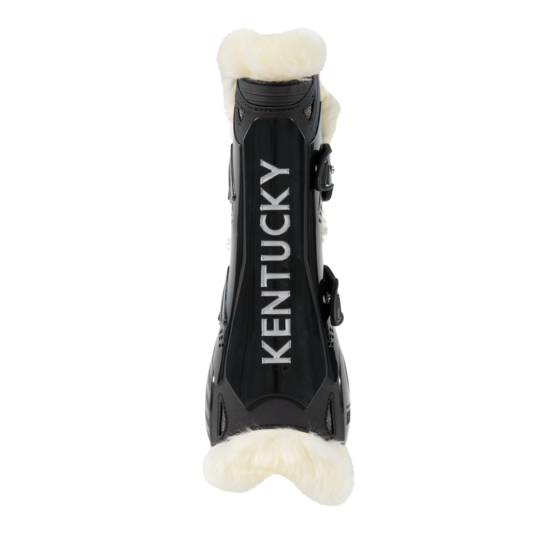The image depicts a black plastic brace, likely a protective device for a horse's leg. The brace features the word "Kentucky" written vertically in light gray or silver letters. It is equipped with white fluffy padding on both the top and bottom edges, ensuring comfort and preventing pain when worn. The right side of the brace has small buckles or straps partially visible, indicating that it can be securely fastened around a limb. The entire device is set against a plain white background, highlighting its sleek and sturdy design intended for leg protection.